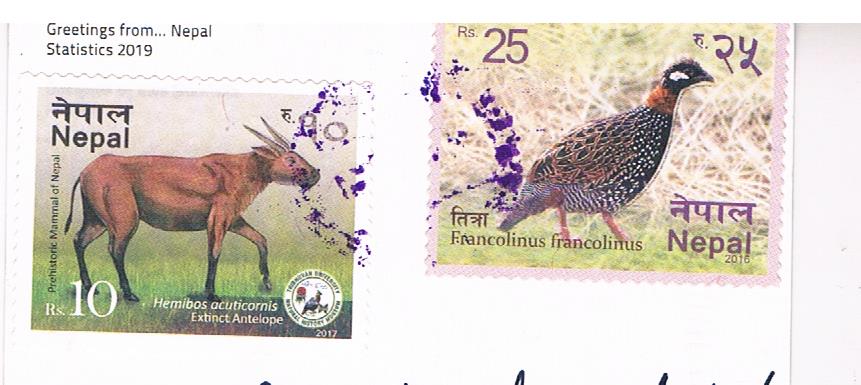The image features two Nepalese postage stamps on a white background with the text "Greetings from Nepal, Statistics 2019" in the top left corner. The left stamp depicts a brown antelope with antlers, standing in grass, and labeled "RS 10." The antelope, a rare and potentially extinct species, is drawn with realistic detail. The right stamp features a bird, specifically a Francolinus, walking on grass with twig-like shrubbery in the background. This bird has a dark body with spotted markings and feathers rimmed with brown, and the stamp is labeled "RS 25" along with "Nepal 2015" in the lower right corner.